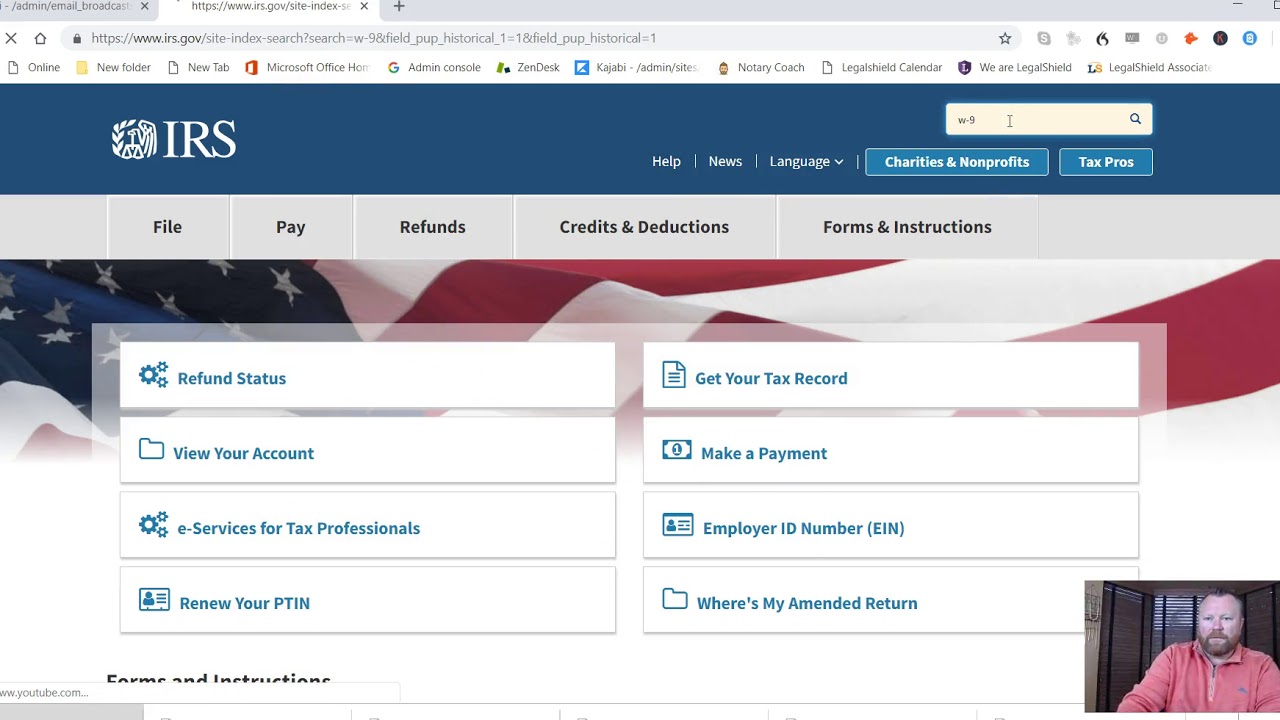This screenshot, taken from a desktop or laptop computer, displays the webpage of the IRS website, as indicated by the address bar showing "https://irs.gov." The IRS logo, distinct in navy blue with the letters "IRS," is prominently displayed. The website's navigation menu includes options such as "Help," "News," "Language," "Charities & Nonprofits," and "Tax Pros." Below, additional menu items like "File," "Pay," "Refunds," "Credits & Deductions," and "Forms & Instructions" are visible.

In the detailed view, specific sections like "Refund Status," "View Your Account," "E-Services for Tax Professionals," "Renew Your PTIN," "Get Your Tax Record," "Make a Payment," "Employee ID Number," and "Where's My Amended Return" are clearly listed.

At the bottom of the screen, there's an inset showing a gentleman with facial hair and fair complexion, wearing an orange shirt, engaging in a screen recording. Behind the IRS website interface is a faint overlay of an American flag, featuring red and white stripes with a blue field of white embroidered stars.

Further desktop elements include icons and labels such as "Online," "New Folder," "New Tab," "Microsoft Office," "Admin Console," and "Zendesk," indicative of the various tools and applications accessible from this desktop.